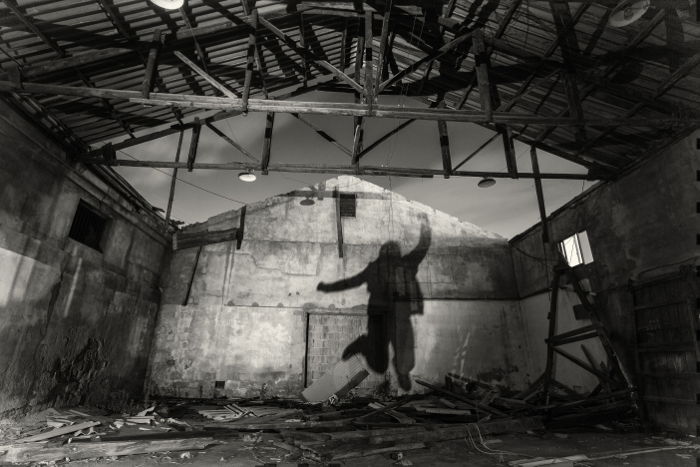This black and white artistic photograph captures the haunting yet evocative interior of a decrepit, partially destroyed building, possibly a barn or warehouse. The image showcases the structure's dilapidated state, with the front half of the roof still intact while the back half has completely collapsed, allowing a gray sky to peek through. The walls, made of concrete and brick, stand in partial ruin, adorned with skeletal beams and broken scaffolding. Scattered across the floor is a chaotic assembly of broken boards, pallets, wood debris, a shattered ladder, and a fallen bookcase, all testifying to the building's abandonment.

A striking feature of the photograph is the back wall, where the light casts a distinct, joyful shadow of a person jumping with one leg kicked up and an arm raised triumphantly, creating a powerful contrast against the bleak surroundings. Small windows and hanging lights contribute to the eerie ambiance, while beams and rusted parts add to the complexity of the scene. The image poetically juxtaposes ruin and elation, capturing a fleeting moment of joy amidst desolation.